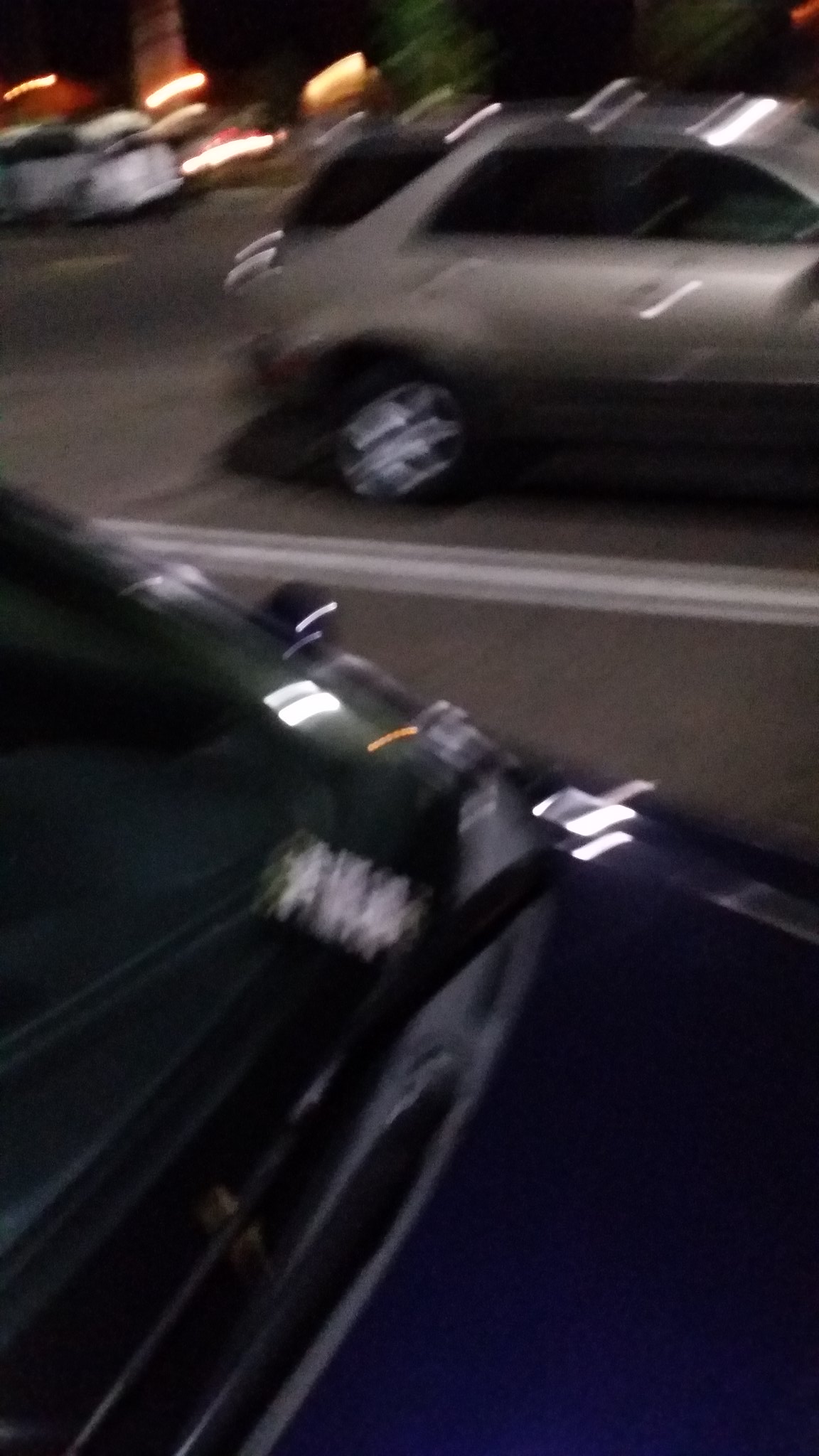This nighttime photograph, taken from over the hood of a blue car, captures a scene within a dimly lit parking lot. The focal point is a blurry silver sedan or small SUV positioned two parking spaces over, featuring lights reflecting off its top and curving edges. Glints of orange light, possibly from nearby businesses like a small restaurant or stores, punctuate the scene against the dark sky. To the left of the silver car is an empty parking slot, followed by a white sedan in the top left corner with additional orange lights visible nearby. The entire image has an unfocused quality, possibly suggesting motion as it was taken, and the ground shows clear white lines marking the parking spaces.